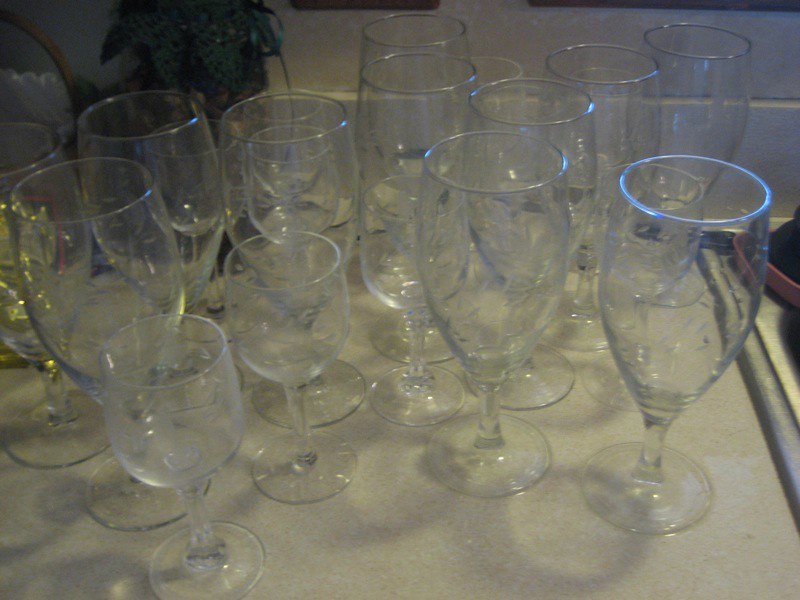A close-up photograph captures an array of clear glassware predominantly consisting of wine glasses and goblets, arranged on a silver tray. The tray, made of shiny metal such as aluminum or steel, occupies the entirety of the frame's bottom section, reflecting the shadows of the glasses. The background, mostly obscured, hints at an indoor setting with a white or light gray countertop visible beneath the tray.

The collection includes approximately 16 to 20 pieces of varying sizes and styles. Some glasses are shorter, with rounded bodies, while others are taller with elongated, cylindrical shapes. A few of the glasses have intricate patterns etched into them. Notably, there is a glass in the front left with a gold foil inside.

Towards the left rear of the arrangement, there appears to be a small brown bucket or vase with a thin wire handle, possibly resembling an ice bucket. Nearby, a green plant or fabric with short leaves is also partially visible. The impression of additional kitchen items, such as a silver-bordered stove, can be seen faintly towards the right side of the image. This meticulous composition highlights the fine details and subtle variety within the glassware, set against an ambient indoor background.